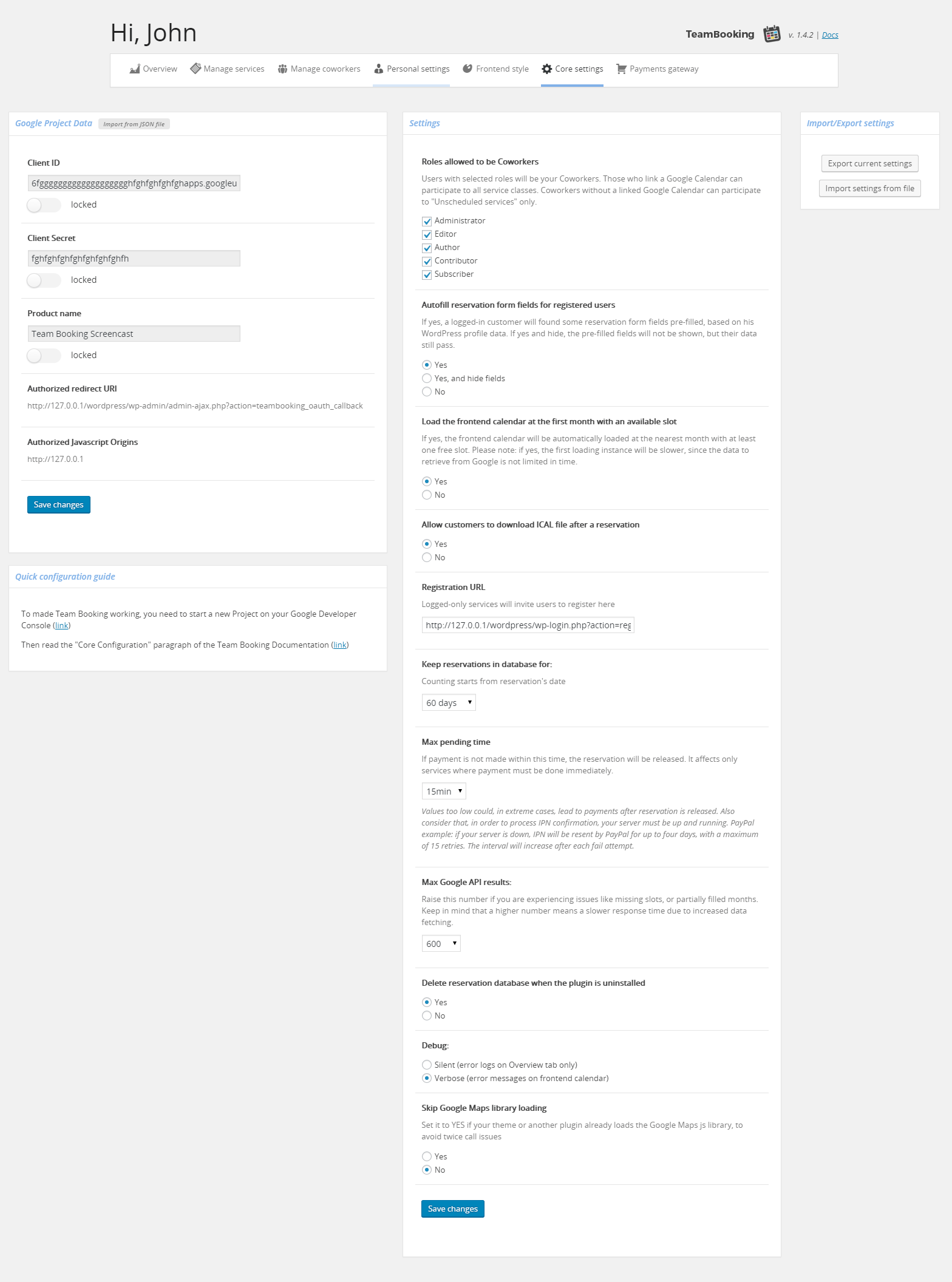The image depicts a potentially problematic screen layout meant for team-building activities. At the top, it says "Hi, John," paired with the phrase "Team-Building" on the right. The screen is cluttered with content divided into what appear to be separate sections, yet the text throughout is too small to read and is in a language other than English. 

On the left side, a full-page segment is split into three sections, each marked by gray bars containing indiscernible symbols. Below this, a blue clickable element and a smaller rectangular section with illegible content can be found.

The right side of the screen showcases two full pages divided into various content blocks. The first page is subdivided into five sections, none of which are readable. The continuation of this page extends into the final section of the image, split into additional sections, and features another blue clickable element at the bottom.

Overall, the screen is densely packed and lacks readability, making it challenging to discern the specific details or intended instructions.